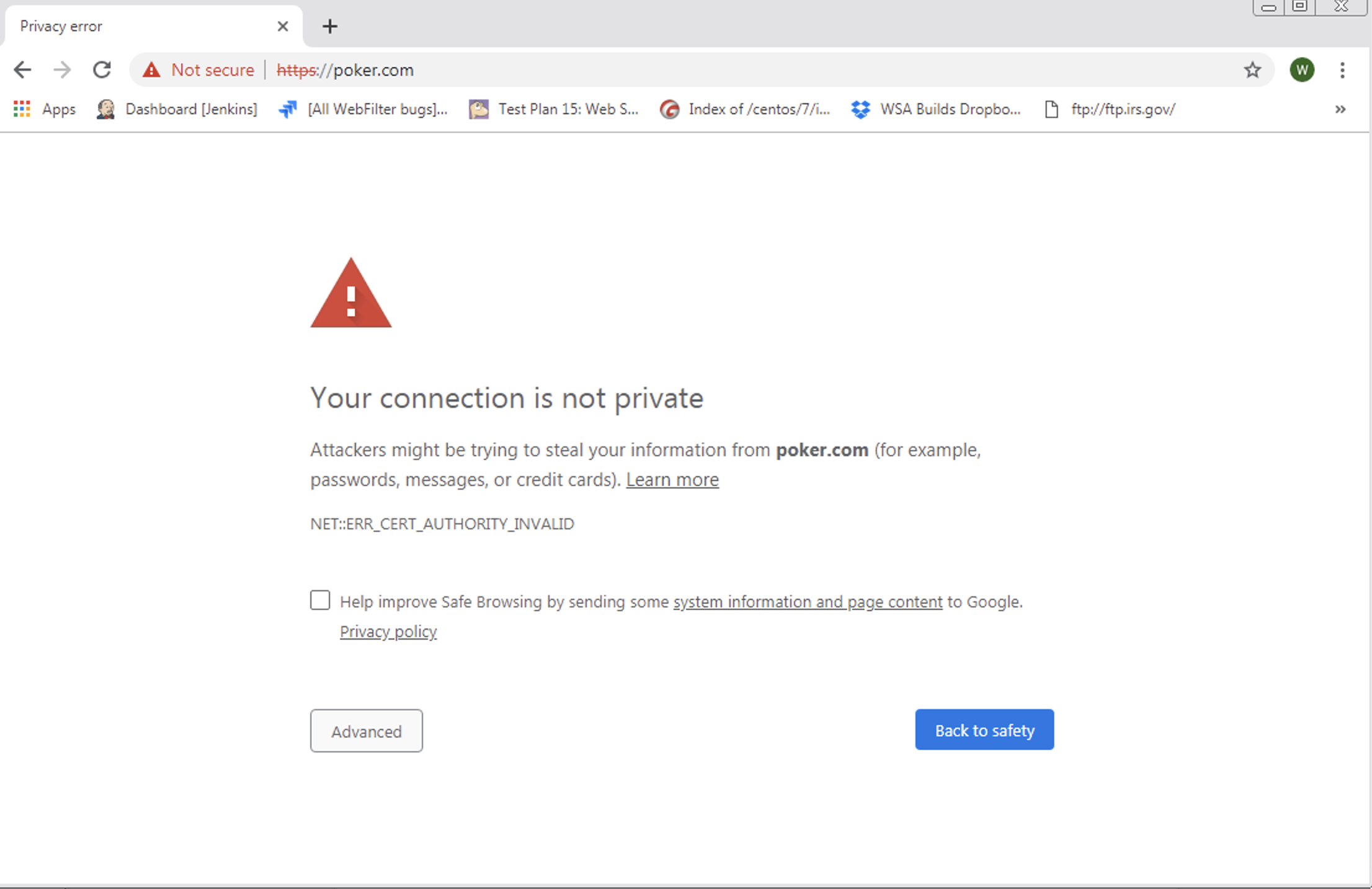The screenshot showcases a computer screen displaying a privacy error warning. The browser window prominently features a "Not Secure" label as the user attempts to access "poker.com." A large red triangle with an exclamation point alerts the user to the critical nature of the issue. The error message states, "Your connection is not private," warning that attackers may be trying to steal information such as passwords, messages, or credit card details. The technical reason given is "NET::ERR_CERT_AUTHORITY_INVALID."

On the screen, there are various other tools and items visible on the dashboard, including a web filter application, a test plan, an index file, and a reference to "WSA bills dropped." Additionally, there appears to be a mention of the IRS among these items.

The privacy error page offers further options: a checkbox to help improve safe browsing by sending system information and page content to Google, a link to the privacy policy, and two interactive buttons. The larger blue button labeled "Back to Safety" encourages users to return to a secure page, while a smaller white button labeled "Advanced" allows users to further investigate or proceed despite the warning.